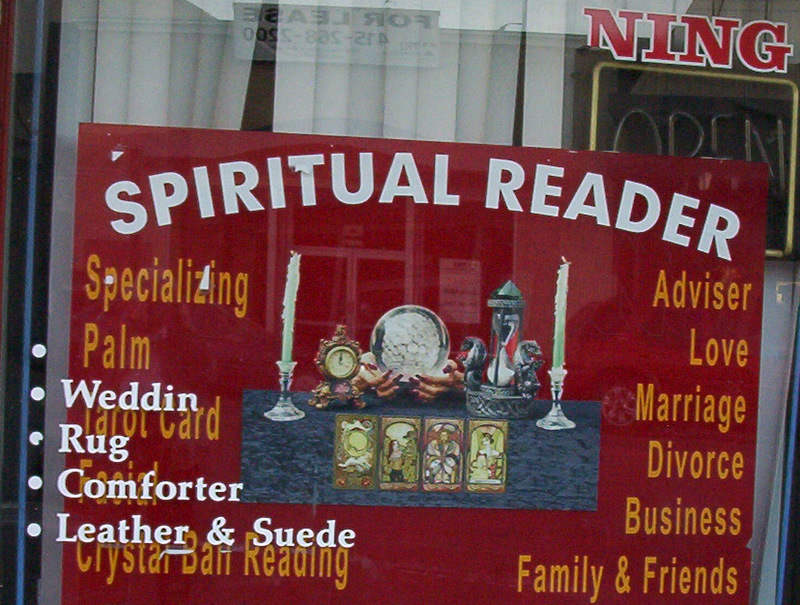This image showcases a storefront advertisement for a spiritual reader, prominently displayed on a glass window with white vertical blinds. The main sign, set against a red background, features bold white letters at the top spelling out "Spiritual Reader." Centrally illustrated on the sign is a table adorned with a crystal ball, candles, and tarot cards, denoting the tools of the trade. Flanking the illustration, the sign details the reader's specializations in gold letters, listing services such as "Palm, Tarot Cards, and Crystal Ball Reading." The right side emphasizes the advisor's expertise in "Love, Marriage, Divorce, Business, Family, and Friends." Additionally, unrelated bullet points on the sign list items like "Wedding, Rug, Comforter, Leather, and Suede." Above the sign, red letters spelling "N-I-N-G" are visible, alongside an unlit open sign.